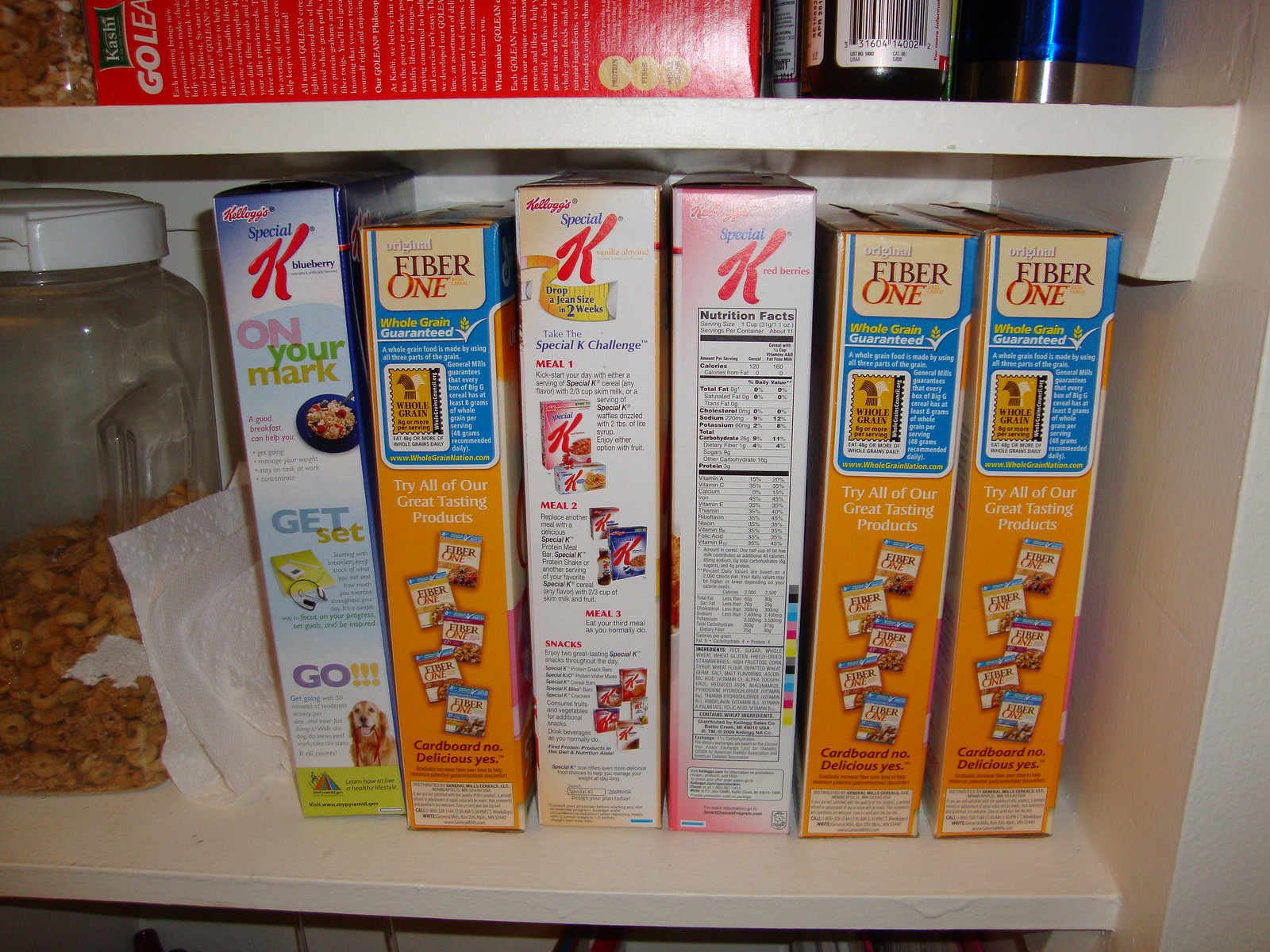The image depicts the interior of a white wooden pantry, focusing on two shelves. The top shelf is partially visible, revealing a Kashi Golean cereal box laid flat, alongside the lower parts of two bottles, one of which has a visible UPC code. The most prominent feature is the lower shelf, which is fully visible and contains six cereal boxes: three boxes of Kellogg's Special K and three boxes of Fiber One, arranged alternately. These boxes are varied in color, including shades of brown, blue, white, and pink. To the left of the cereal boxes sits a transparent plastic container, half-filled with cereal. Additionally, there are individually ripped and folded paper towels next to the cereal on the second shelf. The detailed focus and vibrant colors in the image suggest it's a close-up photograph of someone's well-organized kitchen pantry.